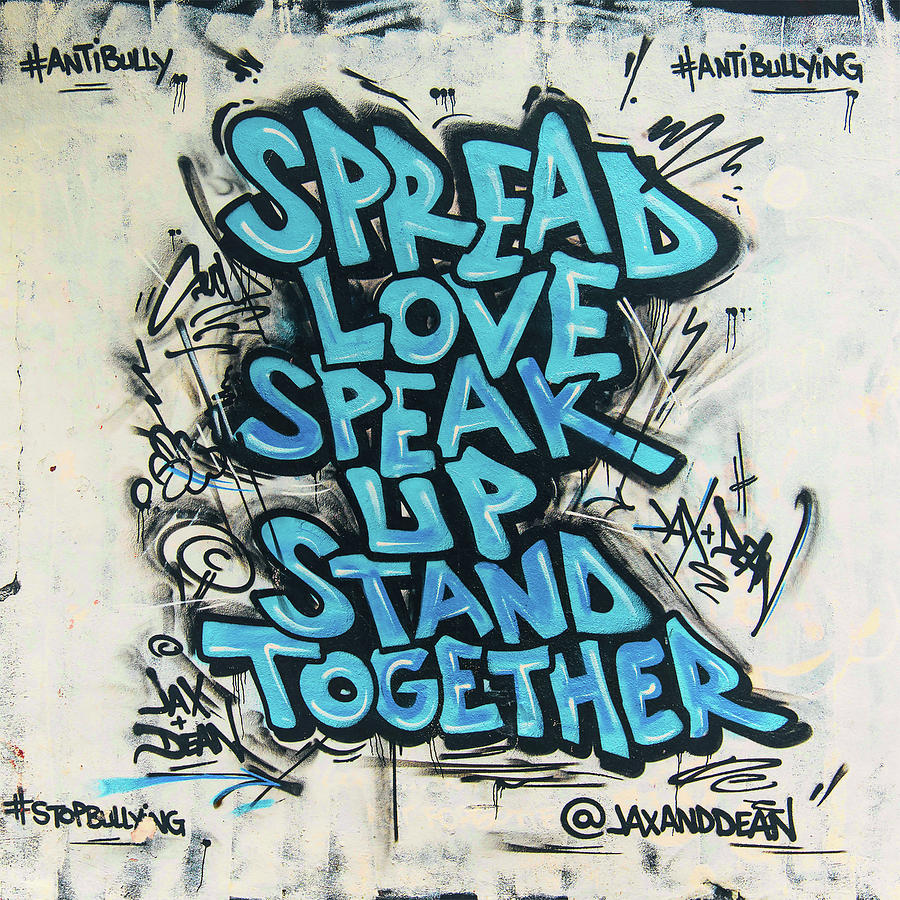This photograph captures a vibrant and powerful graffiti art mural on a white-painted background. The mural features four hashtags prominently displayed in black paint at each corner: "#anti-bullying" in the top left and top right, "#stopbullying" in the bottom left, and the artist's signature "@JaxandDean" in the bottom right. The centerpiece of the mural is a striking message written in large blue bubble letters with white highlights, stating "Spread Love, Speak Up, Stand Together." Surrounding this central message are various accents, including black squiggly lines, exclamation points, and abstract streaks and swirls, giving an impression of dynamic movement and energy. The artists' names, Jax and Dean, appear written twice around the outside of the graphic, adding to the overall sense of unity and collaboration.